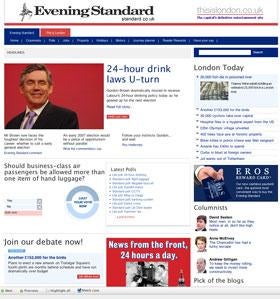Screenshot of a website featuring content from the Evening Standard. The page is divided into two main sections: one highlighted in blue and the other in red. The blue section appears to be the selected or active tab, featuring a header with white text. Below the header, there is an article discussing the 24-hour drink laws. 

On the right side of the blue section, there's a smaller blue rectangle, likely an advertisement, mentioning "heroes" and containing some financial information. Adjacent to it is a red section, which has the headline "News from the Front 24 Hours a Day" and includes profiles of three columnists. Additionally, there is a segment prompting users to "Join Our Debate," providing further details below.